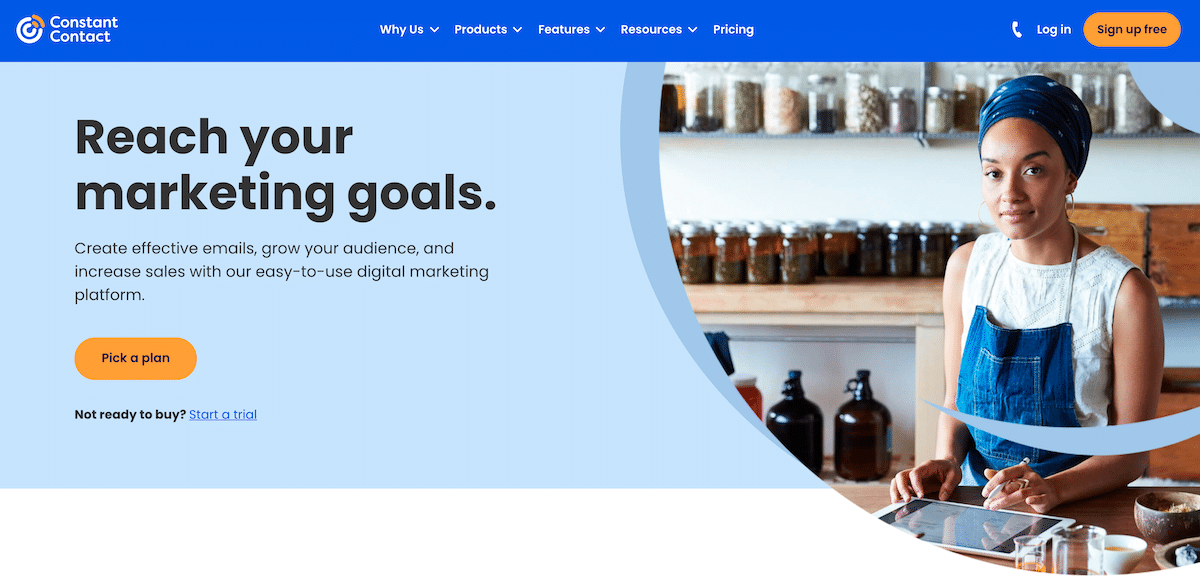This image captures a screenshot of a website landing page for Constant Contact. The top navigation bar, which spans the entire width of the page, is dark blue with white text. On the left-hand side of this bar, the Constant Contact logo is prominently displayed. Centered across the bar are drop-down menu options labeled: Why Us, Products, Features, Resources, and Pricing. To the right, a vibrant yellow button labeled "Sign Up Free" is visible, flanked by a login link and a small telephone icon.

The main body of the webpage has a light blue background with black text. Positioned on the left side, the text reads: "Reach Your Marketing Goals. Create effective emails, grow your audience, and increase sales with our easy-to-use digital marketing platform." Beneath this, an orange button prompts users to "Pick a Plan." For those not ready to commit, there's an adjacent blue hyperlink that says "Start a Trial" next to the text "Not ready to buy."

Dominating the right side of the image is a photograph of a woman wearing a bandana on her head and a sleeveless white blouse, paired with either an apron or overalls. The background shows a set of shelves filled with an assortment of glass jars; clear glass jars are situated on the top shelf, while brown glass containers line the counter. Below these, there are several large dark brown glass growlers typically used for storing alcohol.